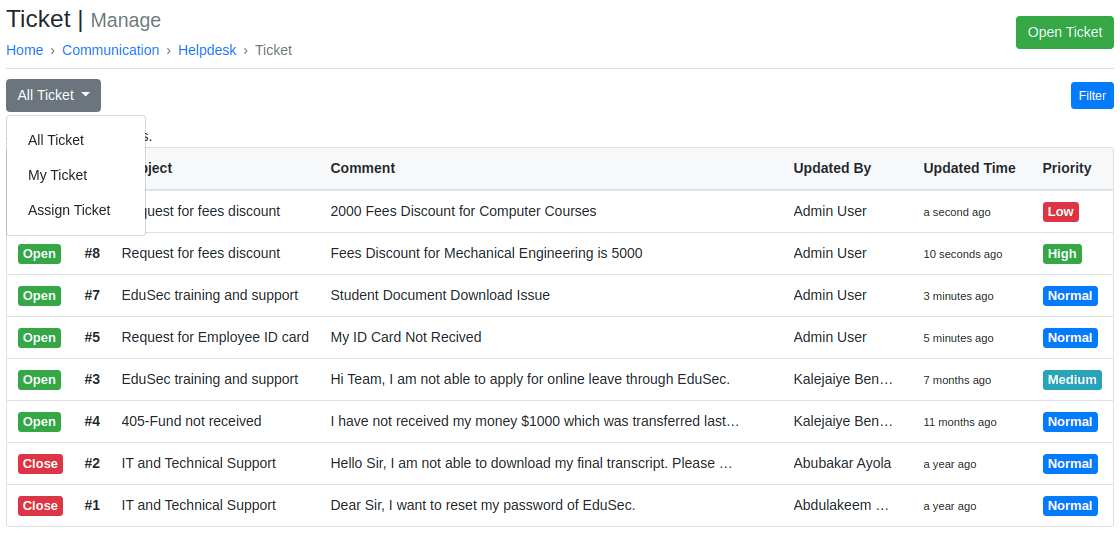The image features a user interface of a Help Desk Ticket Management system. The top section has a white background displaying the text "Ticket Managed Home Communications Help Desk Ticket." Below it, there is a green button labeled "Open Ticket." A horizontal line separates this section from the ticket overview.

Immediately underneath, there is a dropdown menu labeled "All Ticket" in blue, accompanied by a down arrow. This dropdown allows users to filter tickets by categories such as "All Ticket," "My Ticket," and "Assigned Ticket."

The main interface section is organized with columns for "Subject," "Comment," "Updated Time," and "Priority," each highlighted in a light blue box. Here, multiple ticket entries are listed, detailing their statuses and priorities:

1. The first ticket is marked with a red "Low Priority" label.
2. The second ticket indicates a "High Priority" status.
3. Following this, several tickets are flagged as "Normal" in blue.
4. One ticket is marked "Medium" in a lighter blue color.
5. Finally, there are three additional tickets marked "Normal" in blue.

The display shows a total of five open tickets and two closed tickets, with comprehensive details for each entry. This organized layout highlights the functional aspects of the Ticket Manager tool.